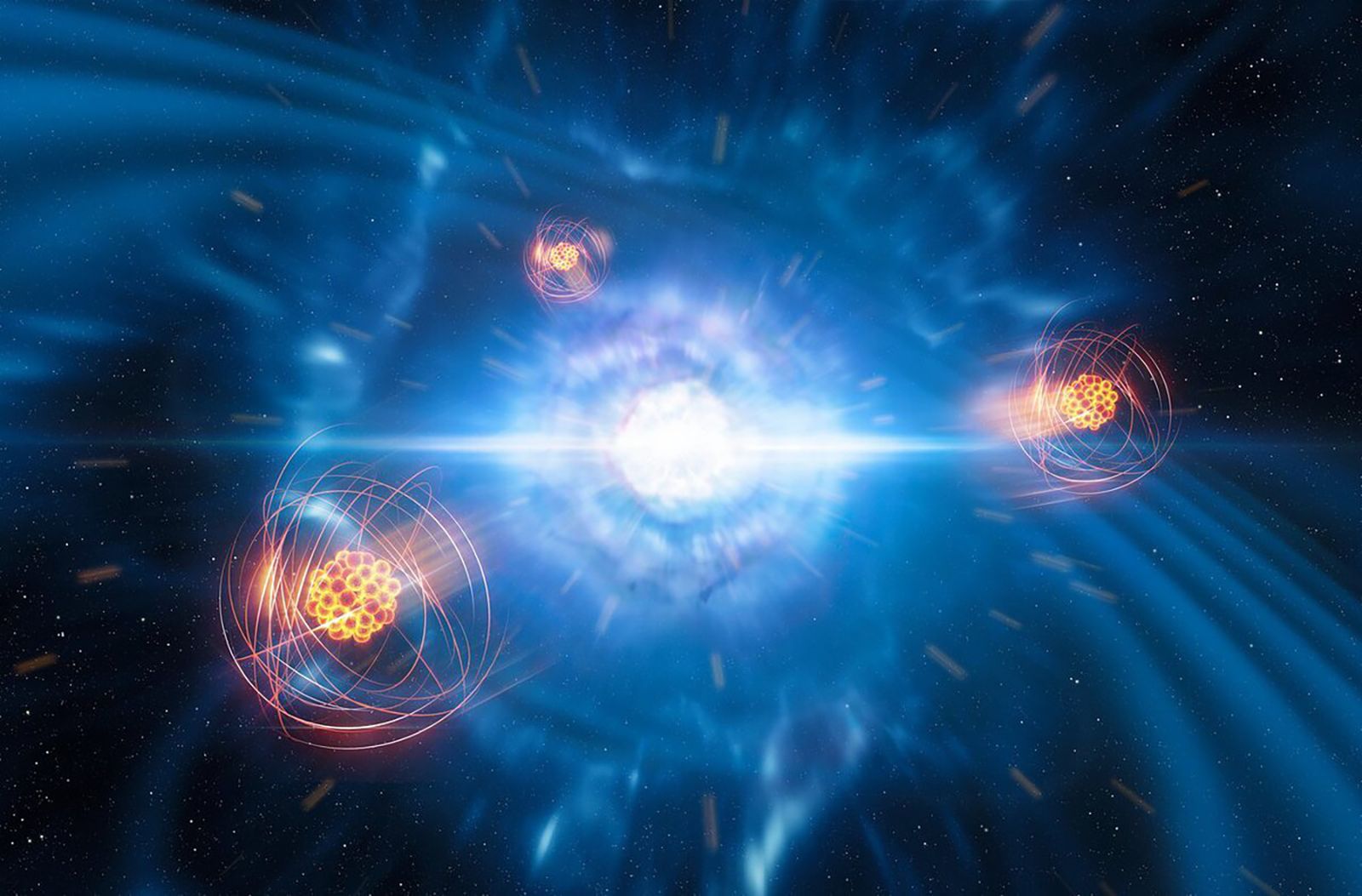In this digital illustration set in outer space, a brilliant star or perhaps a black hole dominates the center of the image, emitting a blinding white and bluish-white light. This central light source displays concentric circular rays, reminiscent of an explosion or intense energy burst, that extend across the dark, star-speckled background. Surrounding this radiant center, three clusters, resembling orb-like formations, are arranged in a triangular pattern. Each cluster is made up of smaller glowing spheres that appear like fiery raspberries, with yellow and orange hues at their cores and streaks of red-orange light circling around them, creating a dynamic, blurred effect as if the image captures rapid movement with a long exposure. The overall scene evokes a sense of cosmic mystery and explosive energy, highlighting the interplay of light and color in the vastness of space.